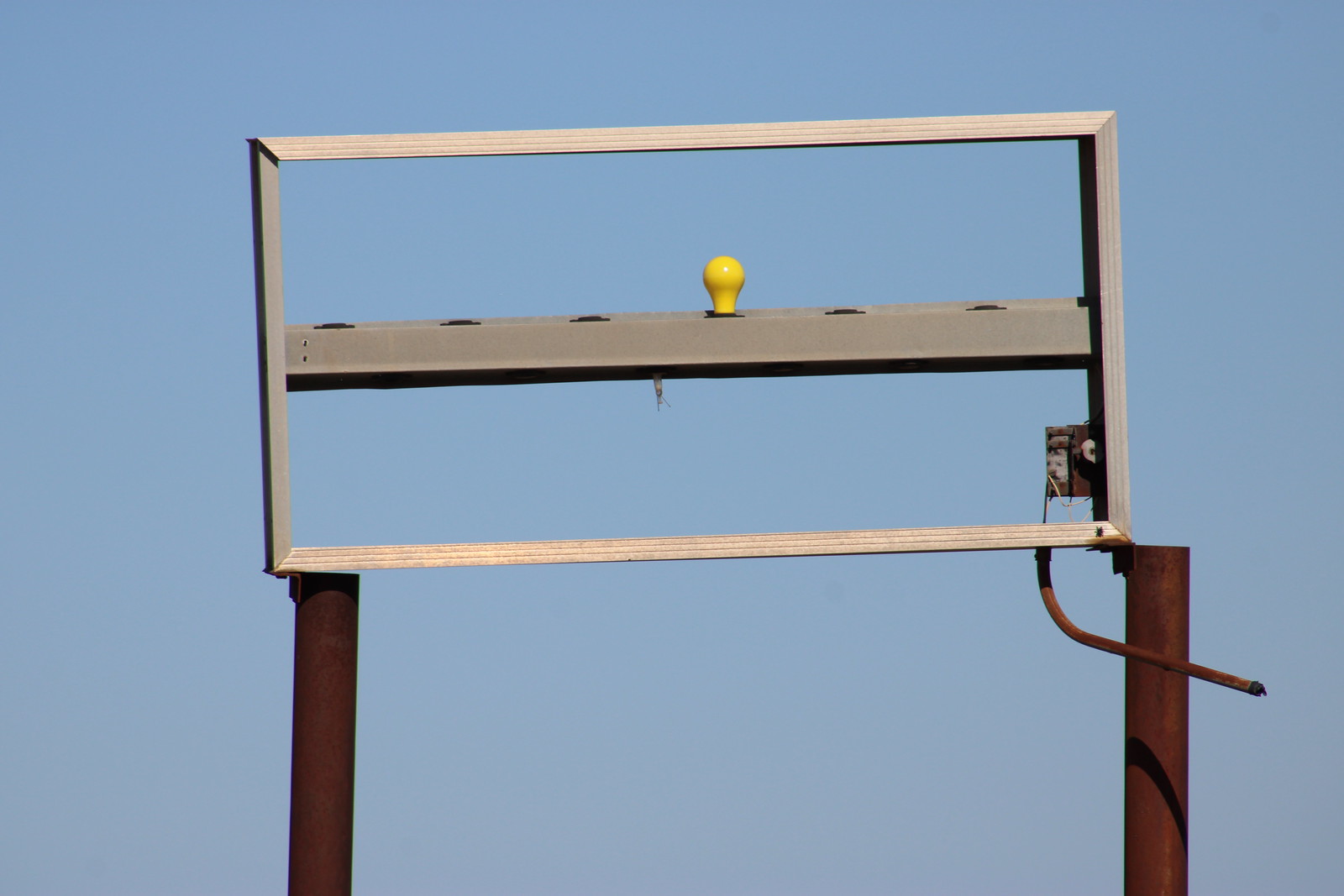This daytime photograph features a clear blue sky backdrop, enhancing the details of an unusual metallic structure prominently displayed in the foreground. At the bottom, two sturdy brown metal posts are visible, with a narrow brown pipe extending from their base. Ascending from the posts, a silver metal rectangle forms the core of the structure. Positioned centrally within this rectangle, a silver metal bar stands out, serving as a platform for several circular indentations. Nestled within these indentations are yellow light bulbs, each entirely yellow and unlit, creating an interesting visual contrast against the metallic elements. The image showcases exceptional quality, capturing every detail with precision. Near the bottom of the silver rectangle, a small, boxy component is mounted within its frame. This component features a mix of brown and silvery hues, adding to the complex and intriguing design of the structure.